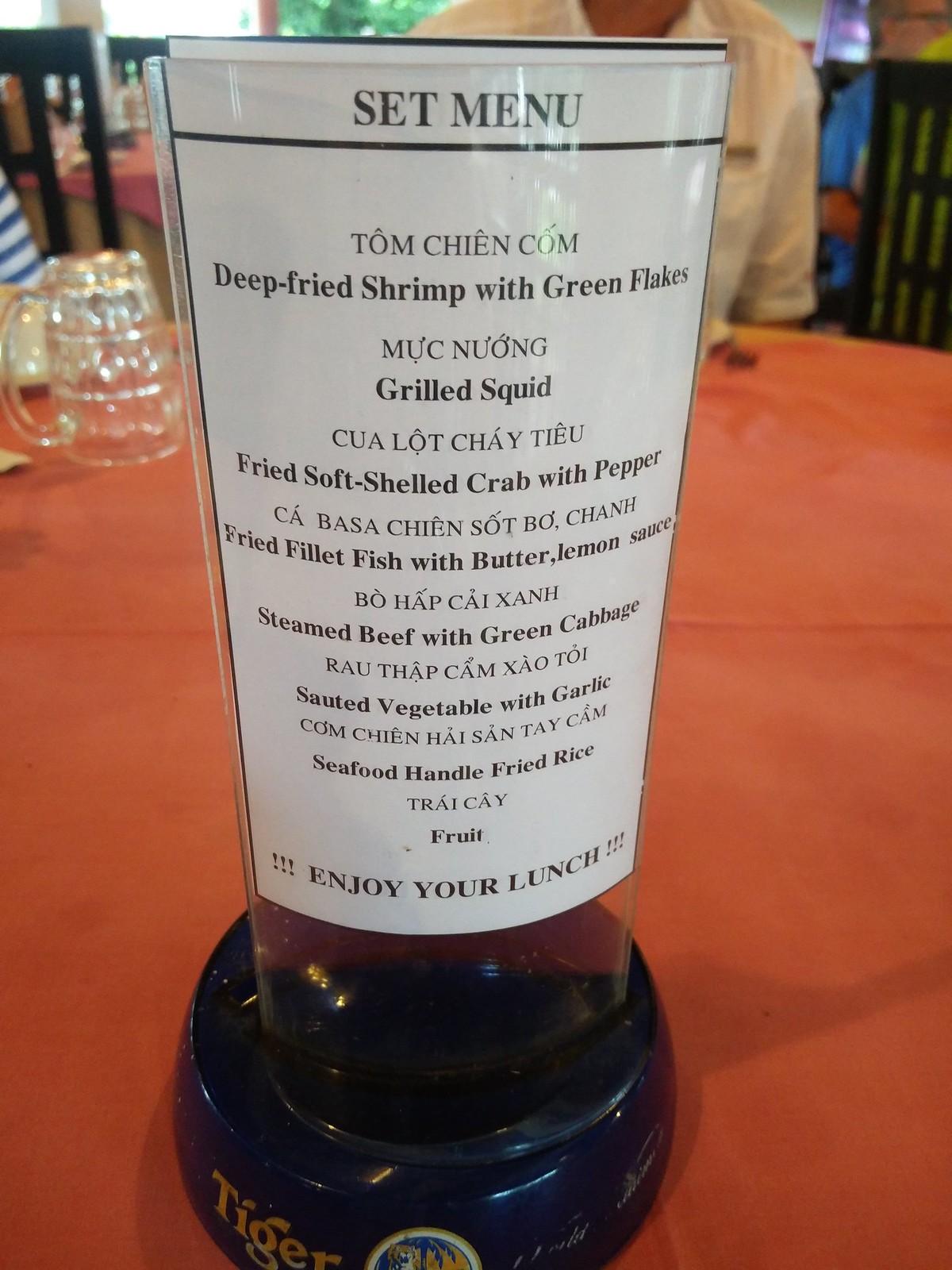The image depicts a detailed restaurant table setting. At the center, there is a glass container functioning as a menu holder. The menu, wrapped snugly around the exterior of the glass, appears to be inserted into a clear plastic sleeve, allowing for easy removal and replacement. This glass container sits on a dark blue base, which prominently features the word "Tiger" in a dark gold, metallic color. Beside the gold text, there is a cursive inscription and a partial emblem, both in the same dark gold hue.

The table itself is draped in a red tablecloth, setting off the colors of the menu holder brilliantly. In the top left corner of the image, a glass mug is positioned upside down, with its handle pointing to the left, adding to the layered and thoughtfully arranged composition of the table setting. The mug contrasts with the glass container, emphasizing the well-organized and inviting atmosphere of the dining area.